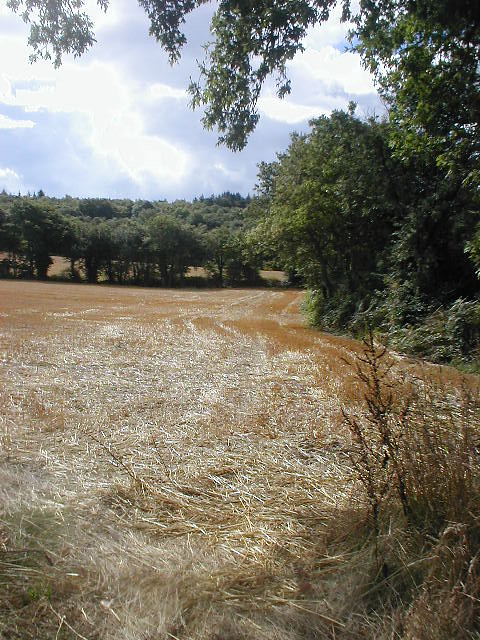This image depicts a sunlit farmland encircled by a dense forest. The bright blue sky, adorned with large white clouds, forms the backdrop. To the left and right, a row of trees extends horizontally, creating a natural border around the field. Closer to the viewer, more trees come into view, with branches and leaves hanging over the top of the image from a tree likely positioned just out of frame to the right. The ground of the field appears to be dirt covered with brown, tamped-down grass and threshed vegetation, suggesting recent harvesting activity. Various shades of brown and tan dominate the field, contrasting with the green of distant trees. At the bottom right, a brown shrub is visible, growing amidst the debris. The entire scene, filled with hues of white, blue, green, black, brown, and tan, captures a tranquil moment in nature, highlighting the interaction between cultivated land and the surrounding forest.